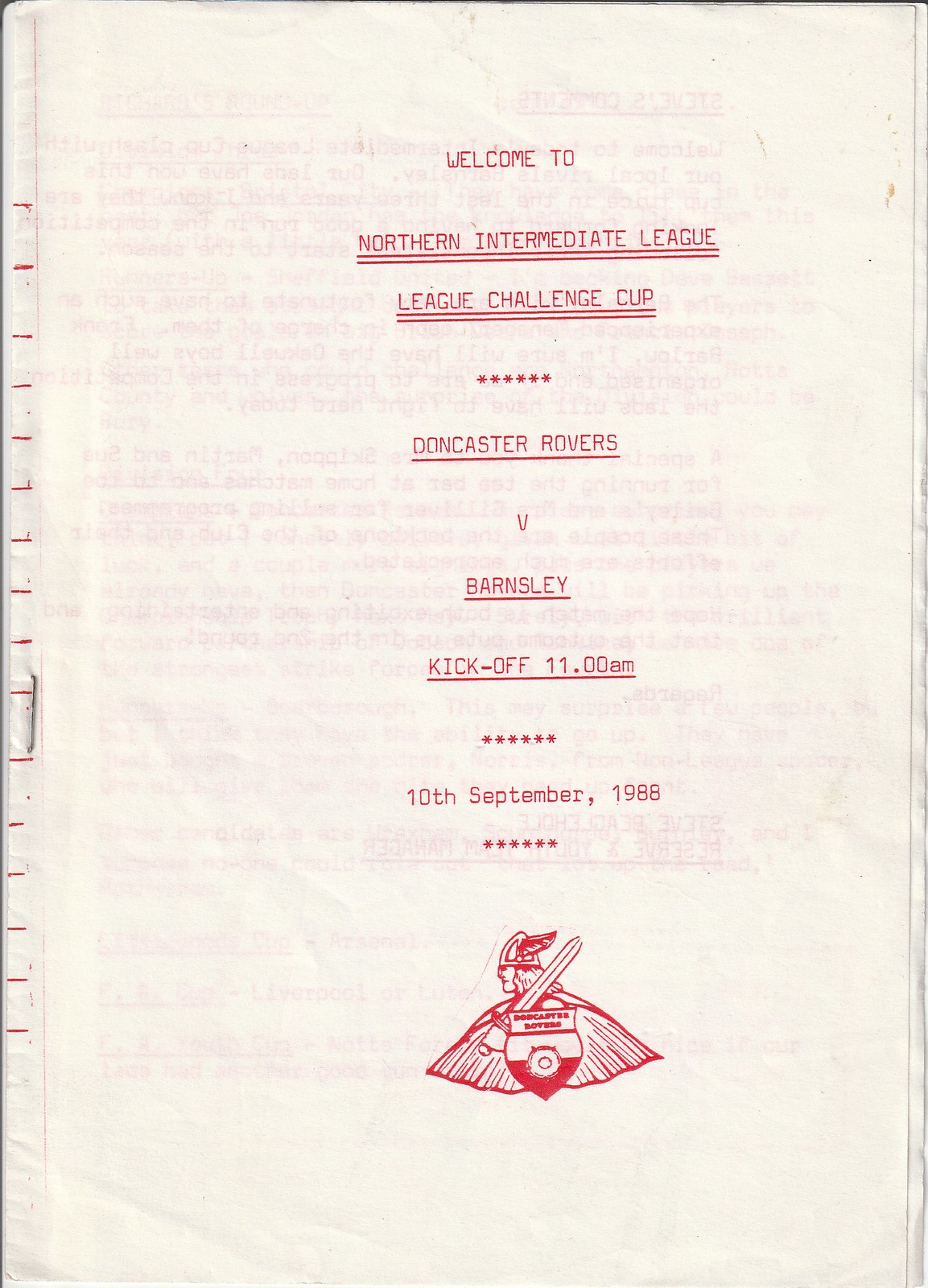The image appears to be the front page of a vintage, low-budget sports program or handbill, likely related to a European football match. The page is an aged, thin white paper, now looking almost beige, and is stapled on the left-hand side, suggesting a DIY magazine or pamphlet. The text is entirely in red and center-aligned. The header reads "WELCOME TO" in all capital letters, followed by "Northern Intermediate League" underlined twice. Below that, it states "League Challenger Cup," also underlined twice. There are six small asterisk stars, then it reads "Doncaster Rovers" underlined, followed by "v. Barnsley," with "Barnsley" underlined. The kickoff time, "11 a.m.," is underlined as well. Another row of six asterisks follows, stating the date, "10th September 1988," not underlined, with another row of six asterisks beneath it. At the bottom of the page, there's a red illustration of a Viking holding a sword over his shoulder, adorned with a cape. A shield emblazoned with "Doncaster Rovers" is also part of the Viking's depiction.